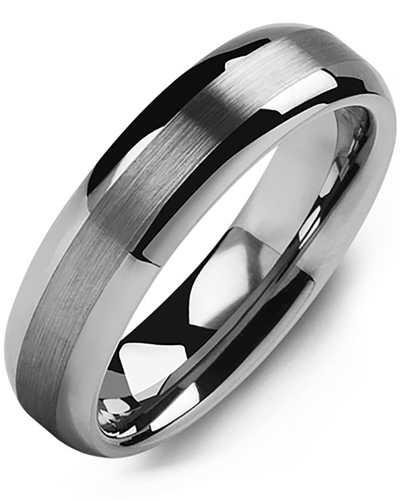This image displays a sophisticated, silver-colored men's wedding ring positioned upright against a stark white background. The exterior of the ring features a dual-tone design with reflective silver on both the top and bottom edges, while a darker, matte silver band encircles the middle, giving a slightly rugged texture compared to the smoother exterior. The interior of the ring is highly reflective, evidenced by two prominent white blotches caused by the reflection of light. The ring's intricate design combines elegant silver hues with a subtle incorporation of darker tones, possibly black or dark quartz, adding a hint of mystique to its appearance. Despite its detailed craftsmanship, there are no text or additional images to provide further context, though its appearance suggests it could also resemble a component of a high-end motorcycle wheel.